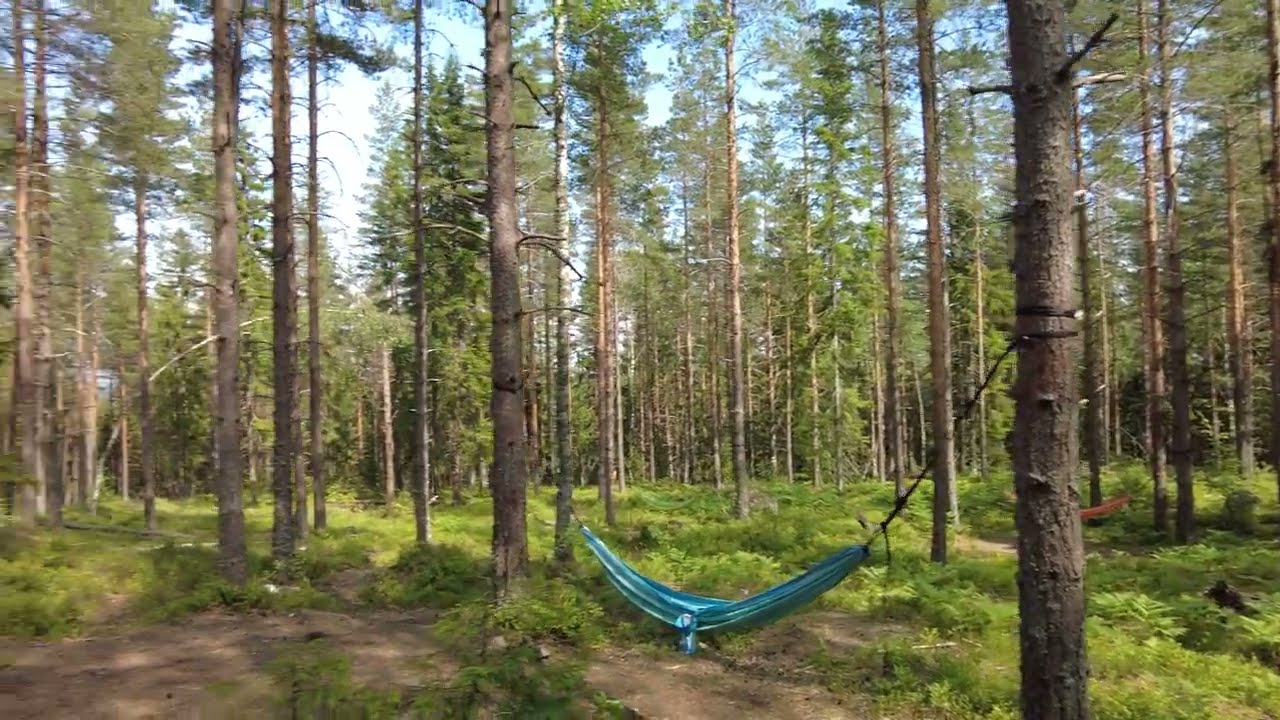The image captures a serene forested area dominated by tall, slender evergreen or pine trees, many of which are nearly limbless up high. The trees are somewhat uniformly spaced, giving a slightly symmetrical appearance, implying they might have been planted intentionally. The terrain underneath consists of both green grass and patches of bare dirt, particularly noticeable in the bottom left and middle regions of the image. A striking feature of the scene is a blue hammock, strung low to the ground between two tree trunks using black ropes. In the background, just behind the blue hammock, a red or possibly tan hammock can be seen faintly tied between another pair of trees. The clear, blue sky overhead hosts a few puffy white or light-gray clouds, bathing the entire area in bright sunlight. Additionally, what seems to be the roof of a building is visible towards the left side of the backdrop.